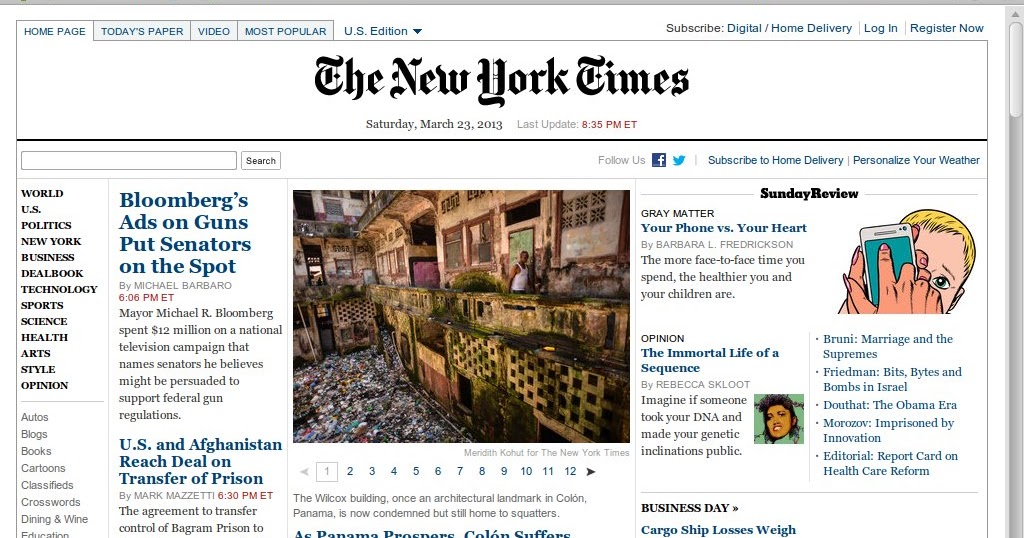Here is a cleaned-up and highly detailed descriptive caption for the image:

---

This image, taken from the New York Times website on Saturday, March 23, 2013, shows a snapshot of the homepage as it appeared last updated at 8:35 PM EDT. At the very top left of the page, navigation links include "Home Page," "Today's Papers," "Videos," and "Most Popular," alongside a dropdown for "US Edition." On the top right, options for "Subscribe," "Digital/Home Delivery," "Log In," and "Register Now" are displayed. A scrollbar along the right edge of the page indicates the currently visible portion of the page—currently at the top.

Below these, a search bar allows users to query the site, and there are buttons to follow the New York Times on Facebook and Twitter, subscribe to home delivery, and personalize local weather updates. The left-hand side of the page features a comprehensive navigation menu with categories such as "World," "U.S.," "Politics," "New York," "Business," "DealBook," "Technology," "Sports," "Science," "Health," "Arts," "Style," and "Opinion." Further down, additional links include "Autos," "Blogs," "Books," "Cartoons," "Classifieds," "Crosswords," "Dining & Wine," and "Education."

Highlighted articles include "Bloomberg’s Ads on Guns Put Senators on the Spot" by Michael Barbaro, posted at 6:06 PM ET, discussing Mayor Michael R. Bloomberg's $20 million national television campaign advocating for federal gun regulations. Another article features U.S. and Afghanistan reaching an agreement on the transfer of control of Bagram Prison, written by Mark Mazzetti and posted at 6:30 PM ET.

In the center of the homepage, a prominent image depicts a man standing on a balcony surrounded by buildings. The caption explains that the Wilcox building, an architectural landmark in Colón, Panama, now condemned though still home to squatters.

To the right of the image, an article titled "Gray Matter: Your Phone vs. Your Heart" by Barbara L. Fredrickson argues that increased face-to-face interaction benefits health for both adults and children. Below this, in the opinion section, "The Immortal Life of a Sequence" by Rebecca Skloot imagines the implications of publicly disclosed genetic information, featured in the Sunday Review.

Further, the page includes brief mentions of articles such as "Brunei, Marriage, and the Supremes," "Friedman Bits, Bytes, and Bombs in Israel," and others covering topics like the Obama era, innovation in Moscow, and a report card on healthcare reform. Finally, a segment titled "Business Day" discusses issues like cargo ship navigation errors.